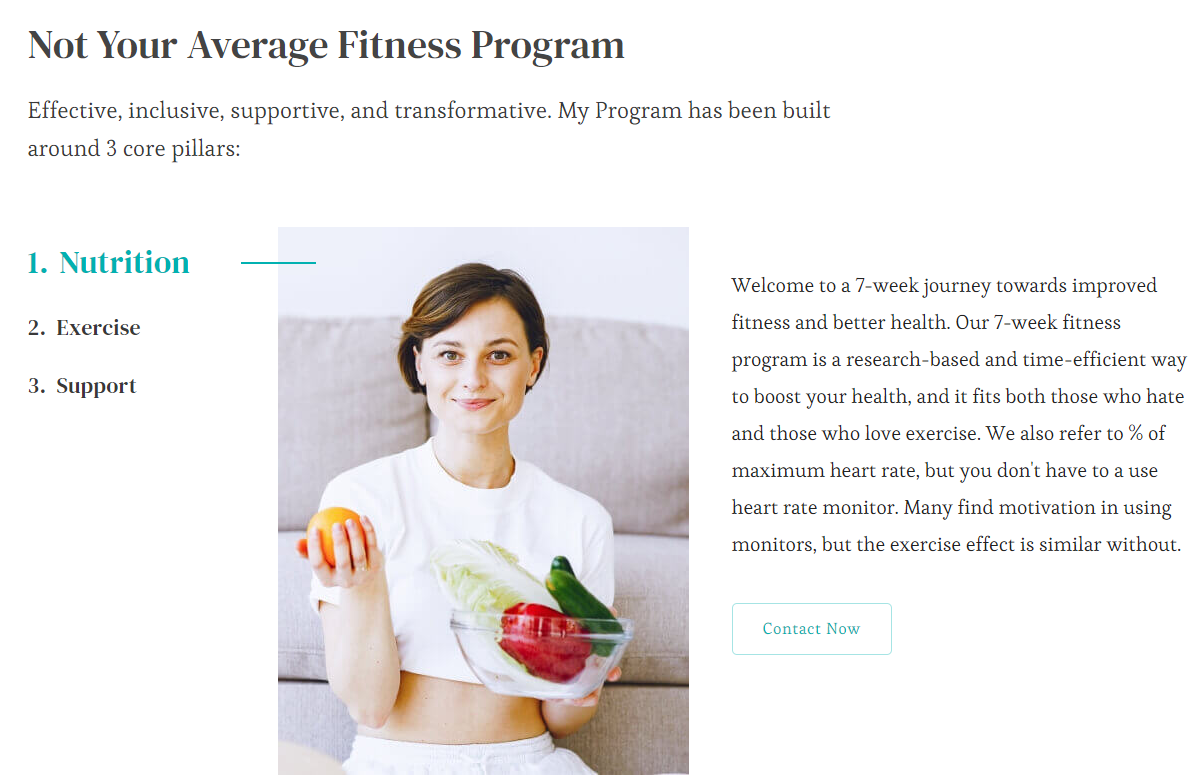Welcome to a transformative seven-week fitness program designed to boost your health in an effective, supportive, and inclusive way. 

The image showcases a smiling woman confidently posing on a tan couch in a cozy living room. She is dressed in a belly shirt and white underwear, holding an orange and two cucumbers, symbolizing the importance of nutrition in our program. The coffee table in front of her displays a clear glass bowl containing a vibrant red pepper and some fresh lettuce, emphasizing the focus on wholesome, balanced meals.

Our program is built around three core pillars: Nutrition, as depicted in the blue letters, Exercise, and Support. The woman's cheerful demeanor highlights the supportive environment we strive to create for all participants, including those in the transgender community. 

In the background, you'll notice the living space's simplicity, featuring a white wall that helps draw attention to the focal points of the image. 

Join us on this seven-week journey towards improved fitness and better health, tailored to participants of all fitness levels. Our research-based approach is designed to be time-efficient and impactful, with or without a heart rate monitor. Start your journey with us today and discover a more confident, healthier you. Contact us now to get started!